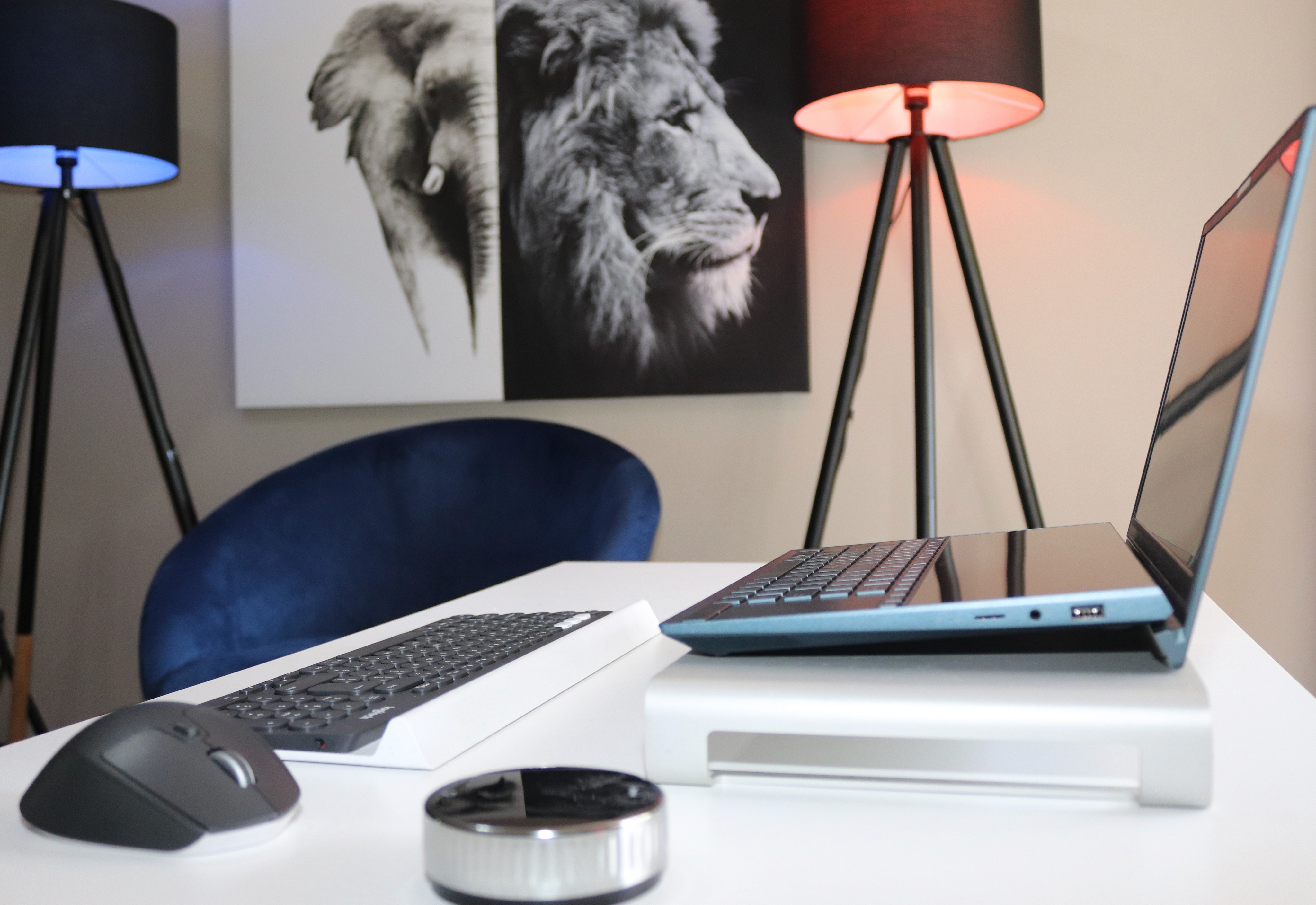The image depicts a sleek and modern office setting with a predominantly monochromatic color scheme, accented by a striking blue chair. Dominating the back wall is a compelling piece of art: a single split canvas featuring a dark elephant on a white background on the left, and a white lion on a dark background on the right. Two tripod floor lamps stand adjacent to the wall, one with a red lampshade casting a warm glow and the other with a blue lampshade emitting a cooler light, both grounded by black frames. 

At the center of the scene is an immaculate white desk. On top of the desk sits a shiny blue laptop elevated on a white riser, flanked by a wireless keyboard and a mouse. An additional object, possibly a sleek stainless steel dispenser, sits to the side, enhancing the modern aesthetic. The dark navy blue, almost royal blue, suede chair positioned at the desk adds a pop of color to this otherwise black-and-white themed office, enhancing the sophisticated and contemporary atmosphere.